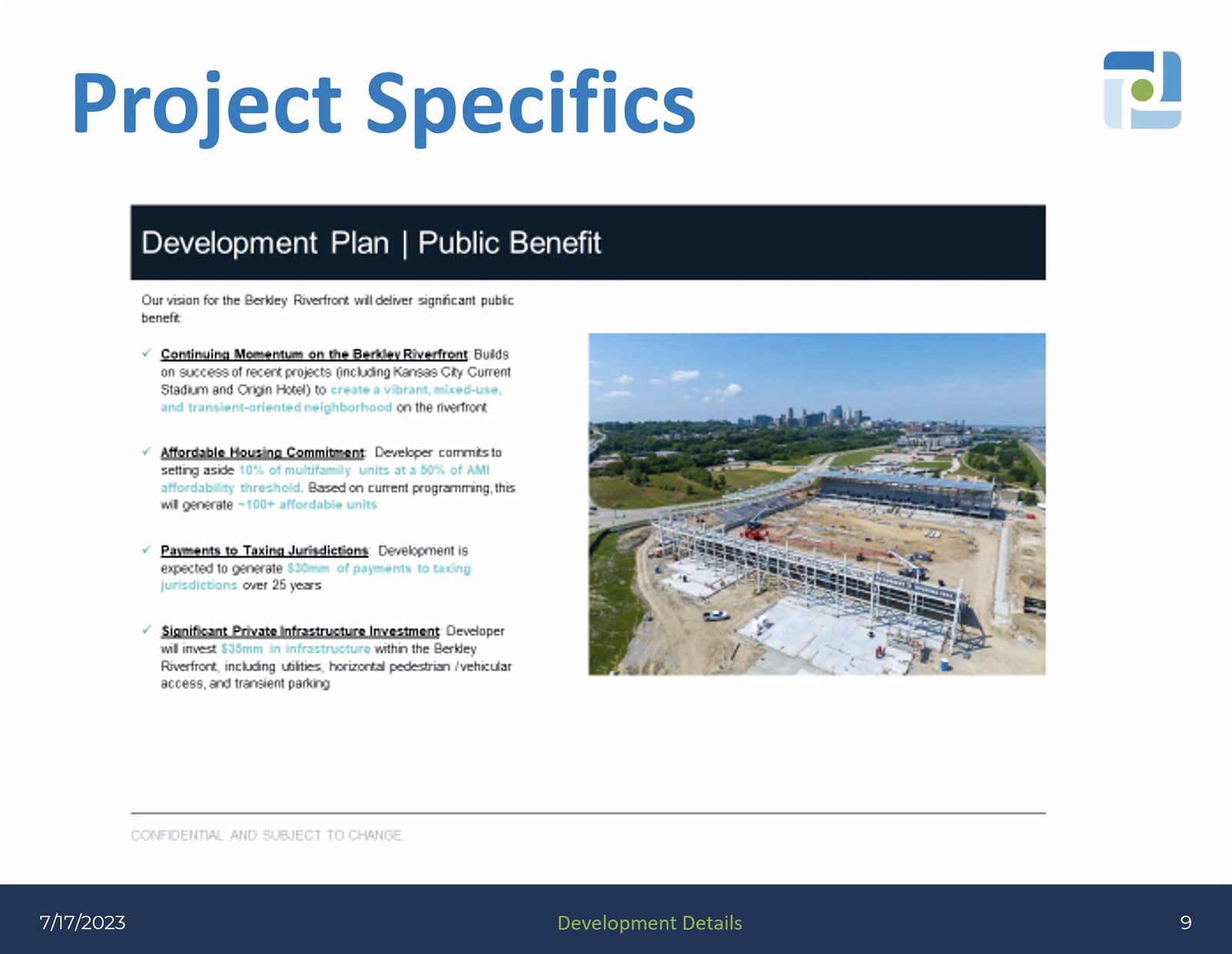The image appears to be a detailed project planning document, possibly a page from a PowerPoint slide or a magazine article. It focuses on the Berkeley Riverhead development, aiming to enhance the Berkeley Riverfront's vibrancy through recent successful projects like Kansas City, Kern Stadium, and the Origin Hotel. The top header, written in large blue font, reads "Project Specifics," and below it, a dark blue bar with white text states "Development Plan / Public Benefit," followed by smaller text in black and light blue detailing the specifics.

Highlighted commitments include setting aside 10% of multifamily units at an affordability threshold of 50% AMI, generating approximately 100 affordable units. The development is anticipated to contribute around $30 million in payments to taxing jurisdictions over 25 years. Additionally, the developer plans to invest $35 million in private infrastructure within the Berkeley Riverfront area, encompassing utilities, pedestrian, vehicle access, and transit parking enhancements.

A photo on the right side depicts a construction site with a partially built structure, a dirt road, surrounding greenery, distant buildings, and blue skies with scattered clouds. The bottom dark blue bar, marked "7-17-2023 Development Details" and "Page 9," underscores the project's contemporary relevance and ongoing development details. The document's overall theme emphasizes the significant public and economic benefits while supporting the Berkeley Riverfront's continued growth. A logo with varying shades of blue and a green circle indicates the document's official nature, while a note mentions that the information is confidential and subject to change.